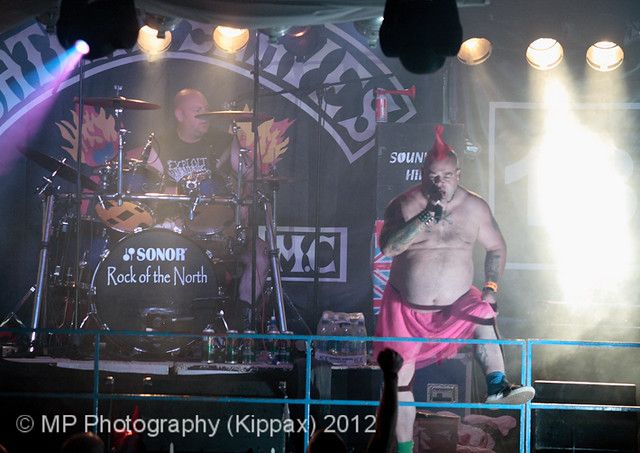In the photograph, we encounter a lively scene from a rock concert, likely of the punk rock variety, set against the backdrop of an energetic stage. The central figure is a portly, shirtless lead singer, exuding charisma and humor with his distinctive pink mohawk standing tall in the middle of his head. He sports a pink skirt, a chain bracelet, and sneakers, with tattoos adorning his arms, and has his right foot propped up on a short, blue railing as he passionately sings into a microphone held close to his mouth.

To the left in the background, a bald drummer is partially visible, engrossed in playing his drum set, which is emblazoned with the words "Sonor, Rock of the North". The drummer is clad in a black tank top that potentially bears the name “The Exploited.” The stage is bathed in the brightness of multiple spotlights, enhancing the concert atmosphere, while a vast black banner with white text looms behind the performers. 

Amidst the bustling concert ambiance, one can also notice decorative flames drawn on either side of the stage. This vibrant moment captured from a distance underscores the dynamic and somewhat whimsical nature of the event. The photograph is marked in the lower left corner with the credit “MP Photography KIPEX 2012,” preserving this snapshot from what appears to be a memorable musical event.